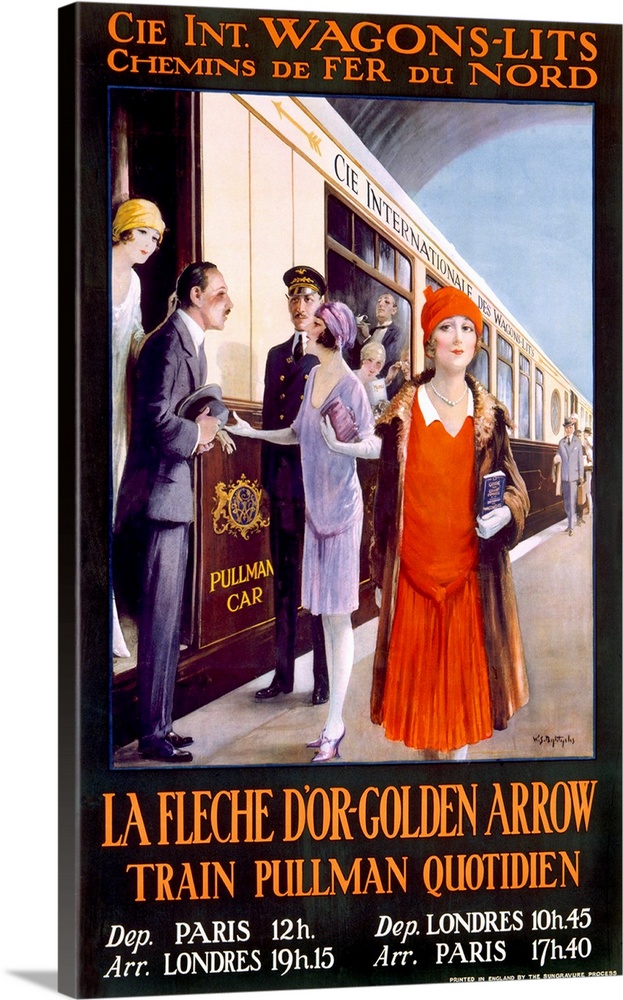The image features a vintage poster, likely from the 1930s or 1940s, advertising the Golden Arrow Train service. This visually captivating piece boasts French text with phrases such as "Chemin de Fer du Nord," "La Flèche d'Or," and "Pullman," indicating its association with the luxurious train service. Prominently displayed are the train departure and arrival times: departing Paris at 12:00 and arriving in London at 19:15, and the return trip departing London at 10:25 and arriving in Paris at 7:40.

Central to the poster is a photograph, meticulously crafted as a graphic depiction, showing passengers at a train station. The scene buzzes with activity as individuals are either boarding or disembarking the train, with notable emphasis on the attire and interactions. In the foreground, a woman dressed in a striking red flapper dress, complemented by a matching red hat and brown coat, gazes directly out of the image, captivating the viewer's attention. Nearby, a man steps off the train, engaging in conversation with another woman, who appears to be greeting him. This intricate portrayal of people, dressed in period attire, truly captures the essence and glamour of the era.